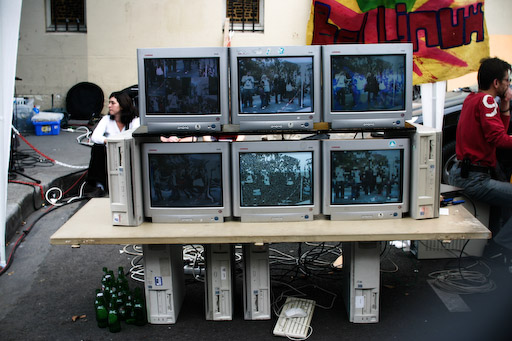This color snapshot photograph, taken outside in landscape orientation, depicts a unique and intriguing setup likely outside a computer service center. Central to the image is a makeshift table composed of a wooden slab, supported by four upright, gray computer towers serving as its legs. Atop the table, six vintage computer monitors are arranged in two horizontal rows of three, each displaying different images. A tangled assortment of electrical cords runs beneath the table, presumably connecting the monitors to the computer towers.

In the foreground, some green glass bottles are scattered under the left side of the table. The background features two individuals: on the left, a Caucasian female in a white long-sleeved shirt with dark hair sits looking to the left; on the right, a Caucasian male wearing jeans and a red long-sleeved shirt with a '9' on the sleeve. He appears to be working, sitting on some kind of machine or crate, and equipped with a walkie-talkie on his black belt. The scene is set against a white building with windows protected by black grating. A colorful hand-painted banner in red, black, green, and pink hues adds a splash of vibrancy to the setting, positioned behind the monitors.